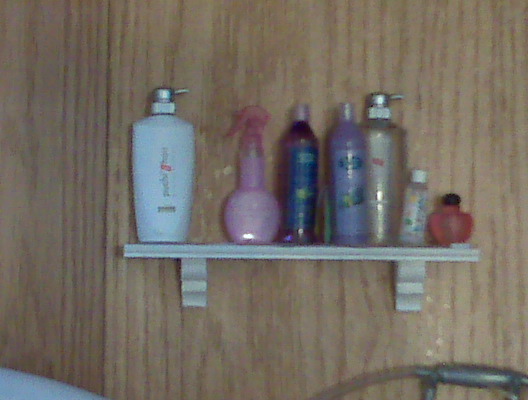In a cozy bathroom, a small white wooden shelf is mounted against a backdrop of warm, light brown wood paneling. This sturdy shelf is supported by two wooden brackets, one on each end, and neatly displays an array of seven colorful beauty products in various shapes and sizes. On the far left, there's a white bottle that appears to be a lotion or shampoo, followed by a pink bottle with an elegant, flowing top. Next, there are two narrow bottles likely containing shampoo or conditioner. Toward the right, a gold bottle with a pump, possibly for skin care, adds a touch of luxury. Completing the arrangement are two small bottles: one clear with floral decorations and one red with a brown top. In the background to the left, the white edge of a bathtub is just visible, while on the bottom right, an indeterminate metal handle slightly protrudes. Interestingly, a little hose peeks out from under the shelf, adding a hint of mystery to the scene.